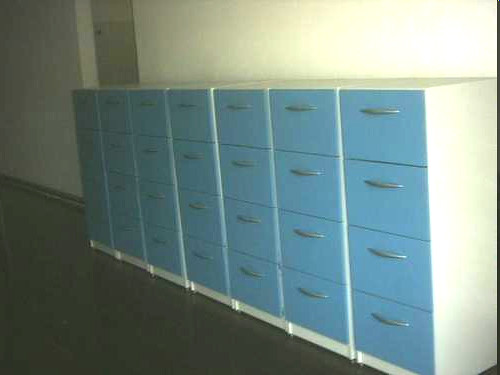The image depicts a series of file cabinets lined up along a wall in what seems to be an office or storage space. The cabinets are arranged in a tight formation, creating the appearance of a single, cohesive unit. There are seven individual cabinets, each featuring four rows of drawers. The drawer fronts are a gradient of baby blue to sky blue, each adorned with a central horizontal handle made of silver-toned metal. The outer casing of these cabinets is a light white or cream color. The wall behind the cabinets is similarly white with a bright light illuminating the right portion of the scene, casting a slight shadow on the left. The floor is a flat, gray color, possibly epoxy, devoid of any line work or detailing, contributing to a clean, modern aesthetic. The entire assembly spans approximately six to eight feet in length, with the tops of the cabinets aligning seamlessly beneath the backdrop of the white wall.